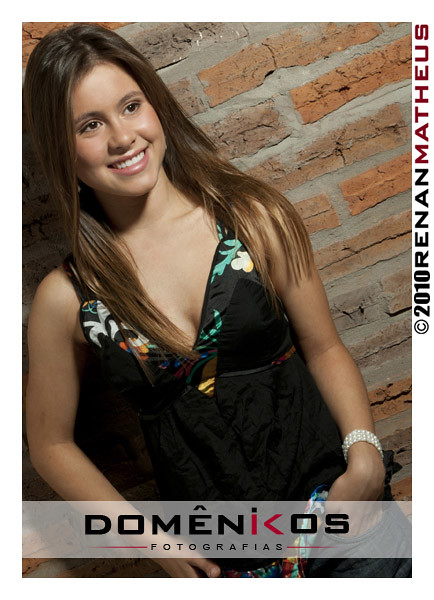The image features a young girl standing against a multi-colored brick wall, primarily composed of red and gray bricks, with prominent cement lines. She is wearing a black, sleeveless, low-cut shirt with green accents and a possible floral print on the shoulder area. A white bracelet adorns her left wrist. Her brown hair falls over one shoulder, and she is smiling brightly, not looking directly at the camera. The photograph has watermarks: "Domenikos Fotografias" near the bottom, and "Copyright 2010, Renan Matheus" in red text on the right side. The setting and lighting suggest the photo could have been taken either indoors or outdoors at night.